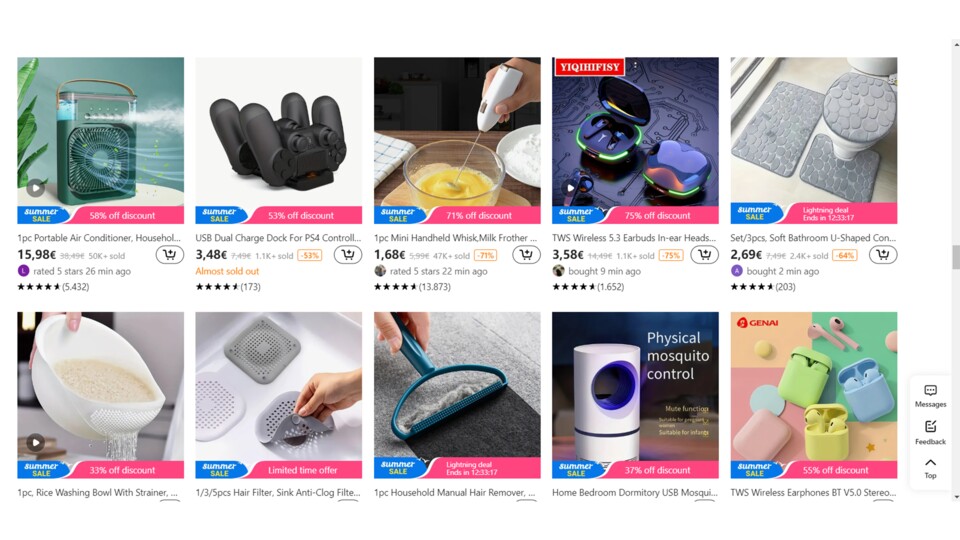Screenshot showcasing 10 home accessories available for purchase on a website, arranged in two horizontal rows of five. Each item is presented with a colorful image and a small blue "Summer Sale" banner. Adjacent to each image, a blue tab-like banner indicates the discount percentage. Directly below each image, a bold one-line description identifies the item, which ranges from portable fans and console game controllers to kitchen utensils, home maintenance accessories, and wireless earphones. The price, listed in pounds, is positioned beneath the description, accompanied by a button with a shopping cart icon to add the item to your virtual basket. Further down, a one-line statement mentions customer ratings and item availability. The final line provides a star rating followed by the number of reviews in parentheses, offering a quick insight into each product’s popularity and quality.